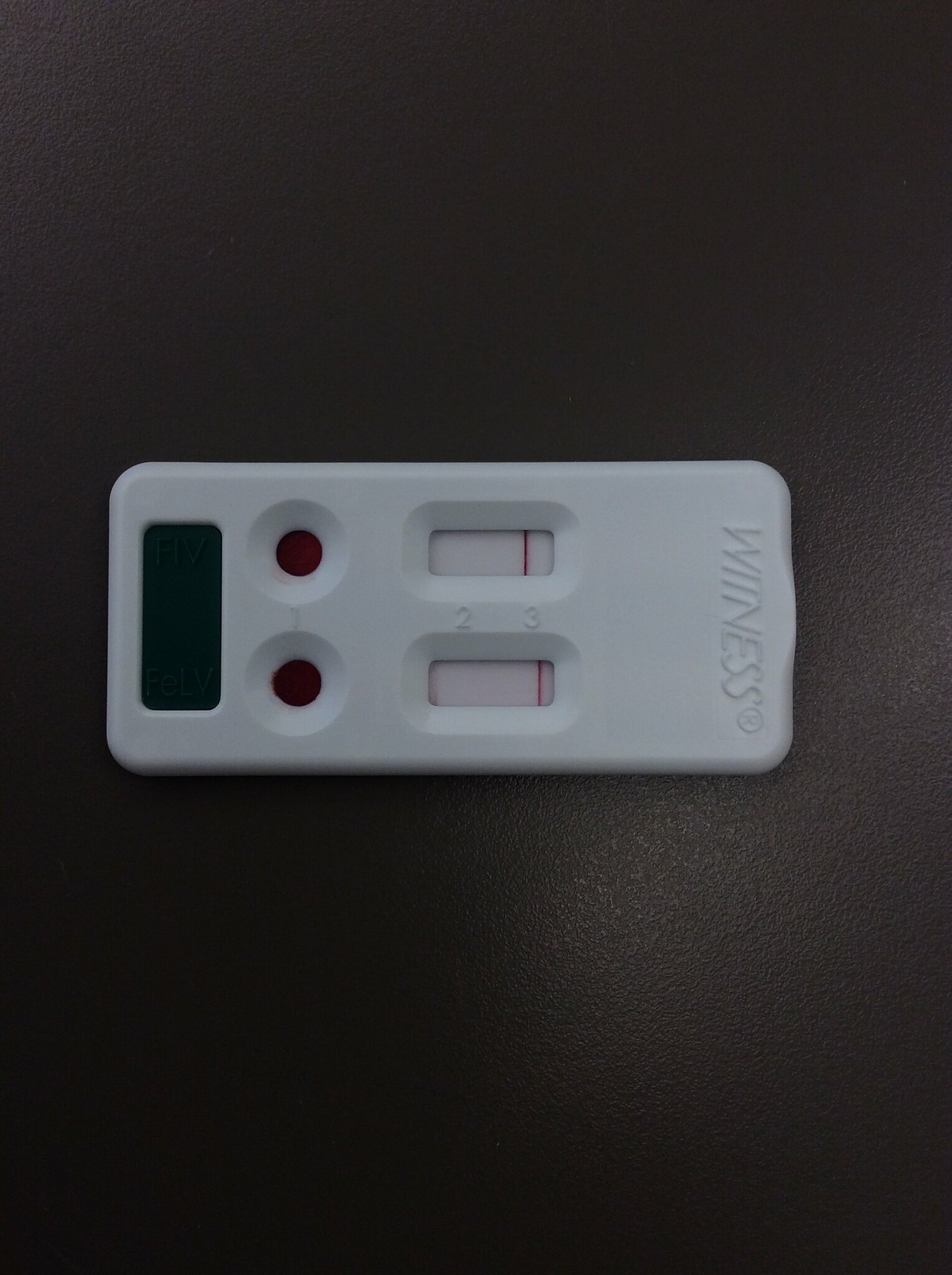The image features a white plastic instrument mounted horizontally on a slightly shiny, gray textured wall. The instrument has a horizontal rectangular shape with rounded edges and is wider than it is tall. On the right side, it bears raised white letters that are difficult to decipher but seem to spell out "WIND," "WINESS," or possibly "WELLNESS." 

In the middle section of the instrument, there are two recessed rectangles, each marked by a vertical red line. Between these recessed areas are the raised numbers "2" and "3." 

To the left of these recessed rectangles, two recessed circles are present, each with a dark red center. On the far left side of the instrument, a recessed green rectangle is oriented vertically. Inside this green rectangle are the raised letters "FIV" and "FELV."